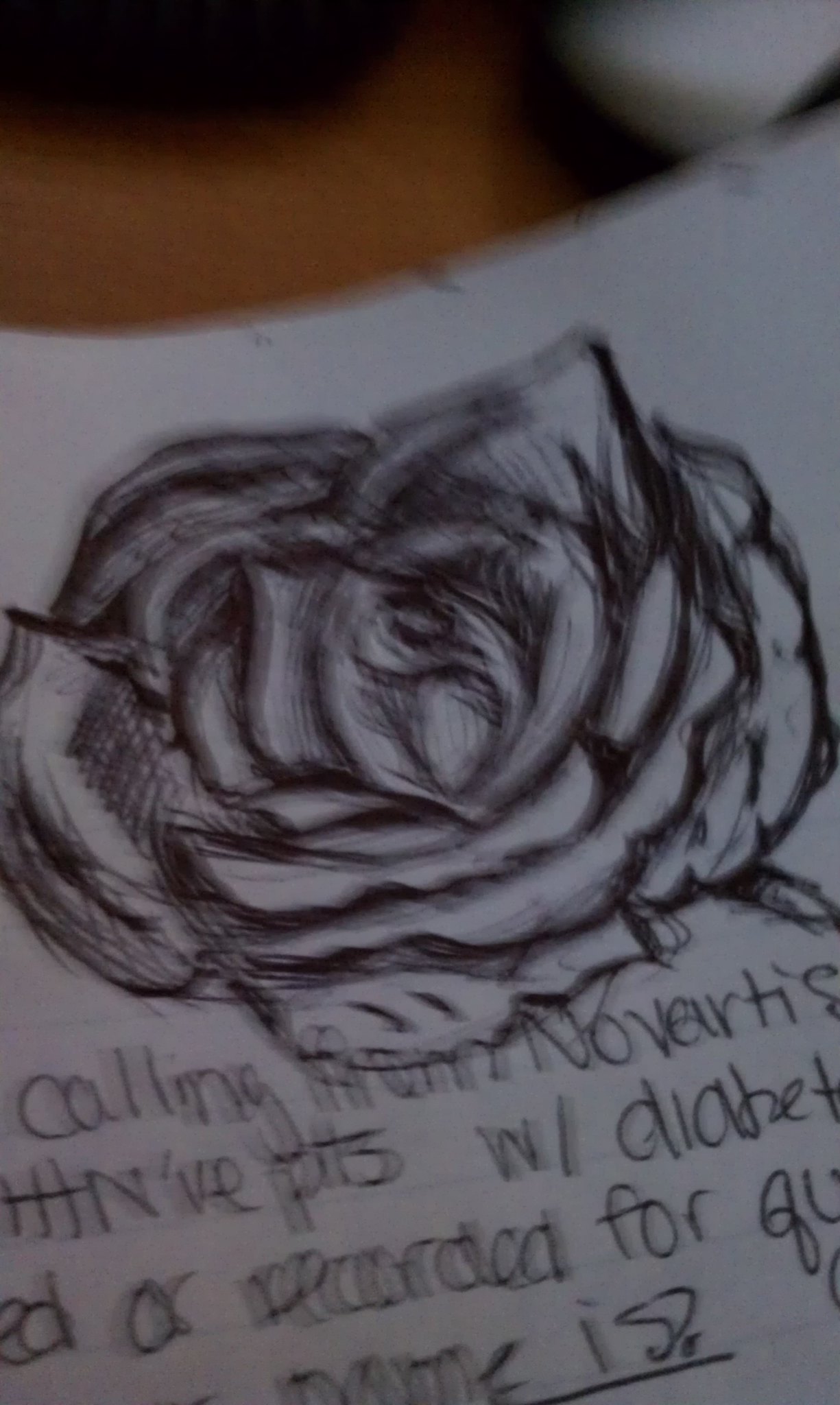A somewhat blurry, portrait-aligned photograph shows a piece of white paper on a brown, possibly wooden table. The paper features a hand-drawn outline of a rose at the top, sketched in black ink or pencil, with some shading to suggest different textures within the flower. Below the drawing is handwritten text in printed letters, though it's difficult to read due to the blurriness and partial cut-off. Some decipherable words include "Calling from Novartis," "PTS," possibly "Patients," with "W / Diabetes," and the word "Recorded." There is also mention of a "Name" with a question mark, suggesting that these may be notes or a doodle, potentially for someone making or reviewing calls related to diabetes patients. The setting includes an unidentified small white object and a shaded black area near the paper.